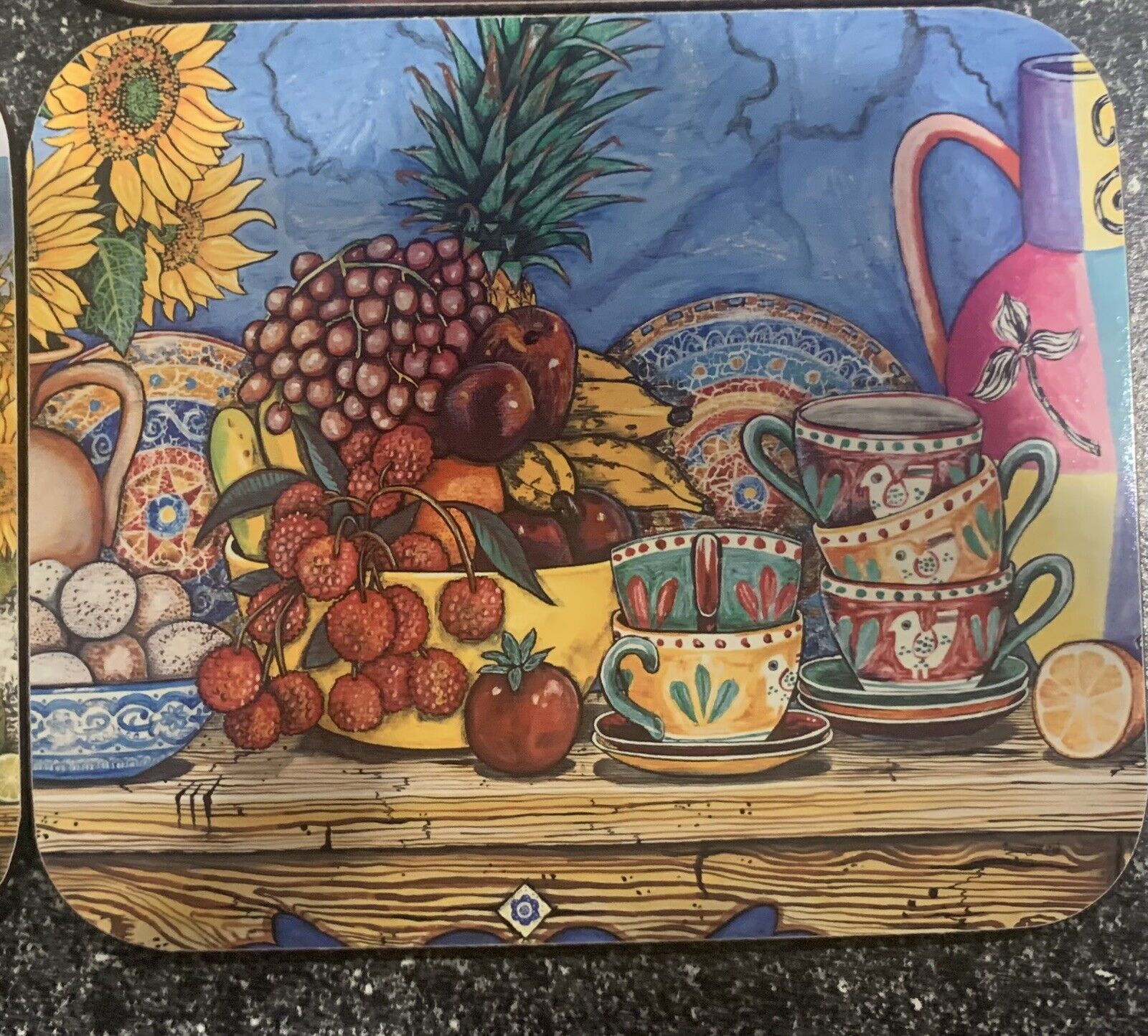This image, which appears to be either a flat tray, a placemat, or perhaps a coaster, rests on a dark granite countertop with specks of white. The artwork is rectangular with rounded corners and features a vibrant, hand-drawn scene. It depicts a wooden table, displaying a variety of colorful items. On this table, there are multicolored teacups, each with green handles, stacked in groups of three and two, accompanied by matching plates. Beside the teacups sits a yellow bowl brimming with an assortment of fruit, including lychees, apples, grapes, bananas, oranges, and a pineapple in the background. Additionally, there's a blue and white artistic bowl containing what appear to be eggs, and nearby, a half lemon and a tomato are visible. In the upper left corner of the image, a vase of bright yellow sunflowers with green leaves adds to the lively scene. Behind this table setting, the background showcases a blue wall with a marbled effect and decorative plates, enhancing the colorful and possibly Latin American-inspired aesthetic of the artwork.